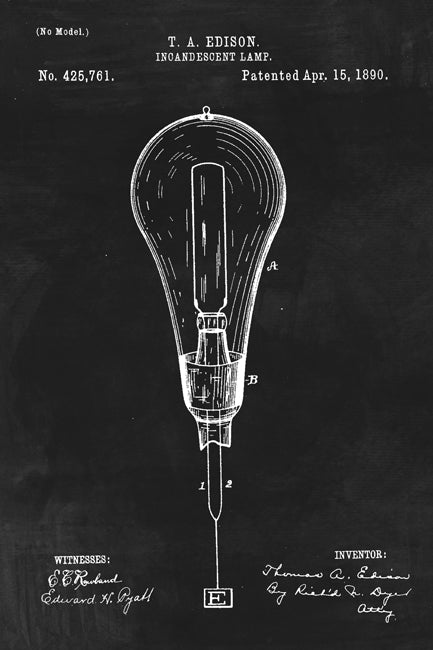This striking illustration depicts Thomas Edison's patented incandescent lamp, rendered in chalk-like white ink on a contrasting black background, giving it the appearance of a blueprint or infographic. At the top left corner, the phrase "No model" is parenthesized, and beneath it, the title "T.A. Edison Incandescent Lamp" is prominently displayed. Below the title, on the left, is the patent number "425,761," and on the right, the patent date "April 15, 1890." Central to the illustration is a detailed diagram of the light bulb, meticulously labeled with various parts marked by numbers and letters such as 1, 2, A, B, and E. The bottom section of the image includes two areas of text: "Witnesses" on the left, accompanied by two signatures, possibly "Edward N. Graft" and "E.G. Rowland," and "Inventor" on the right, attributed to "Thomas A. Edison" with an additional notation crediting "Richard M. Dougall, Attorney." This detailed patent illustration not only highlights the technical elements of Edison's groundbreaking invention but also provides a historical reference to the key individuals involved in the patent process.